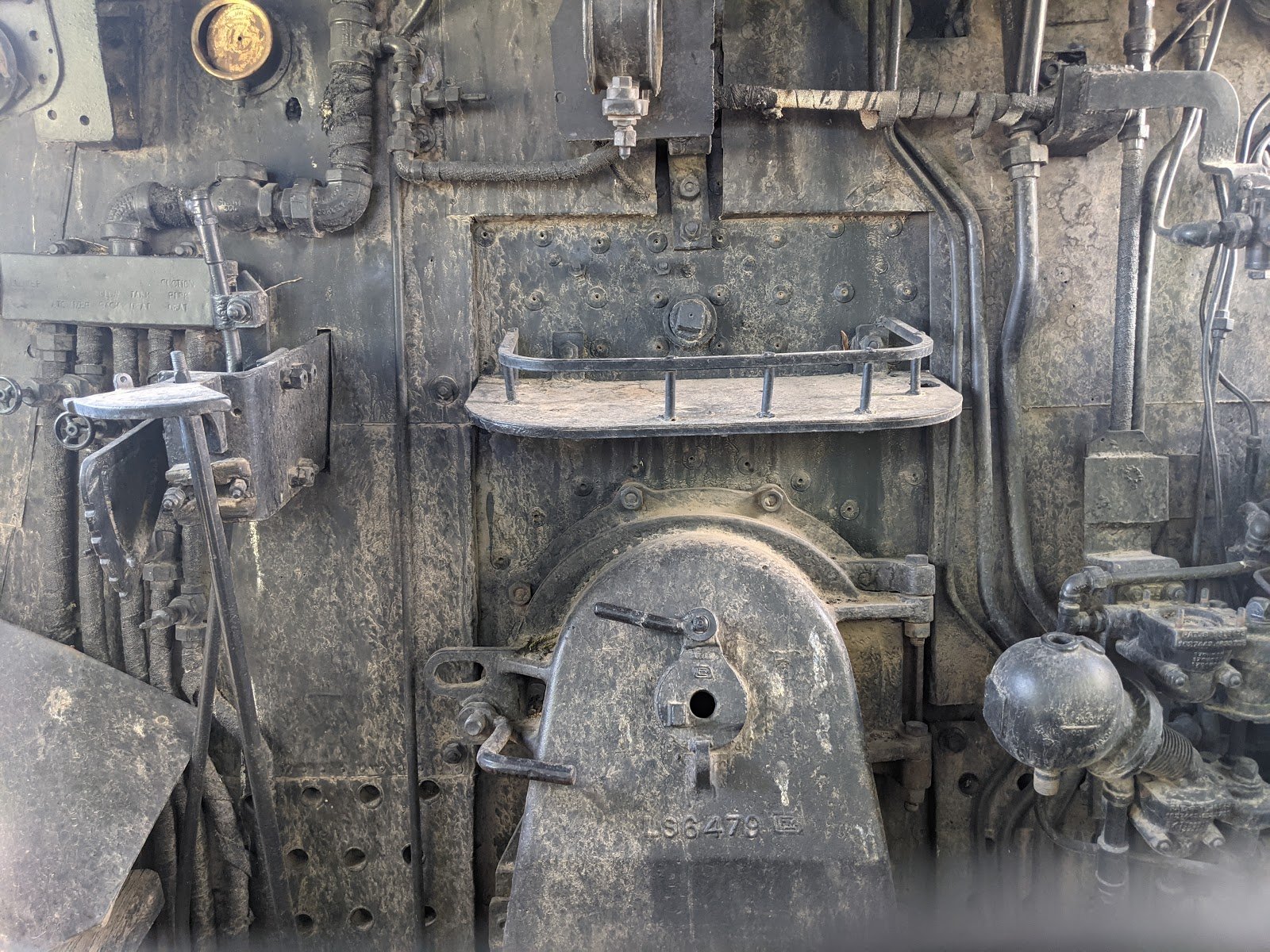The image depicts a very old, dusty steam locomotive covered in gray metal with patches of rust and dirt. At the front of the locomotive, there is a small tray enclosed by a metal fence and an arch-shaped door below it, labeled with the letters "LS6479." To the right of this door, there is a distinct black ball-shaped component connected by a pipe extending to the lower part of the locomotive. The locomotive is adorned with various mechanical elements including gauges, pipes, hoses, brackets, metal wires, and what appears to be release valves. The overall scene suggests a piece of machinery that has long been exposed to the elements, potentially in a ship’s hull or an abandoned train yard, with its metal surfaces corroded and weathered from time.